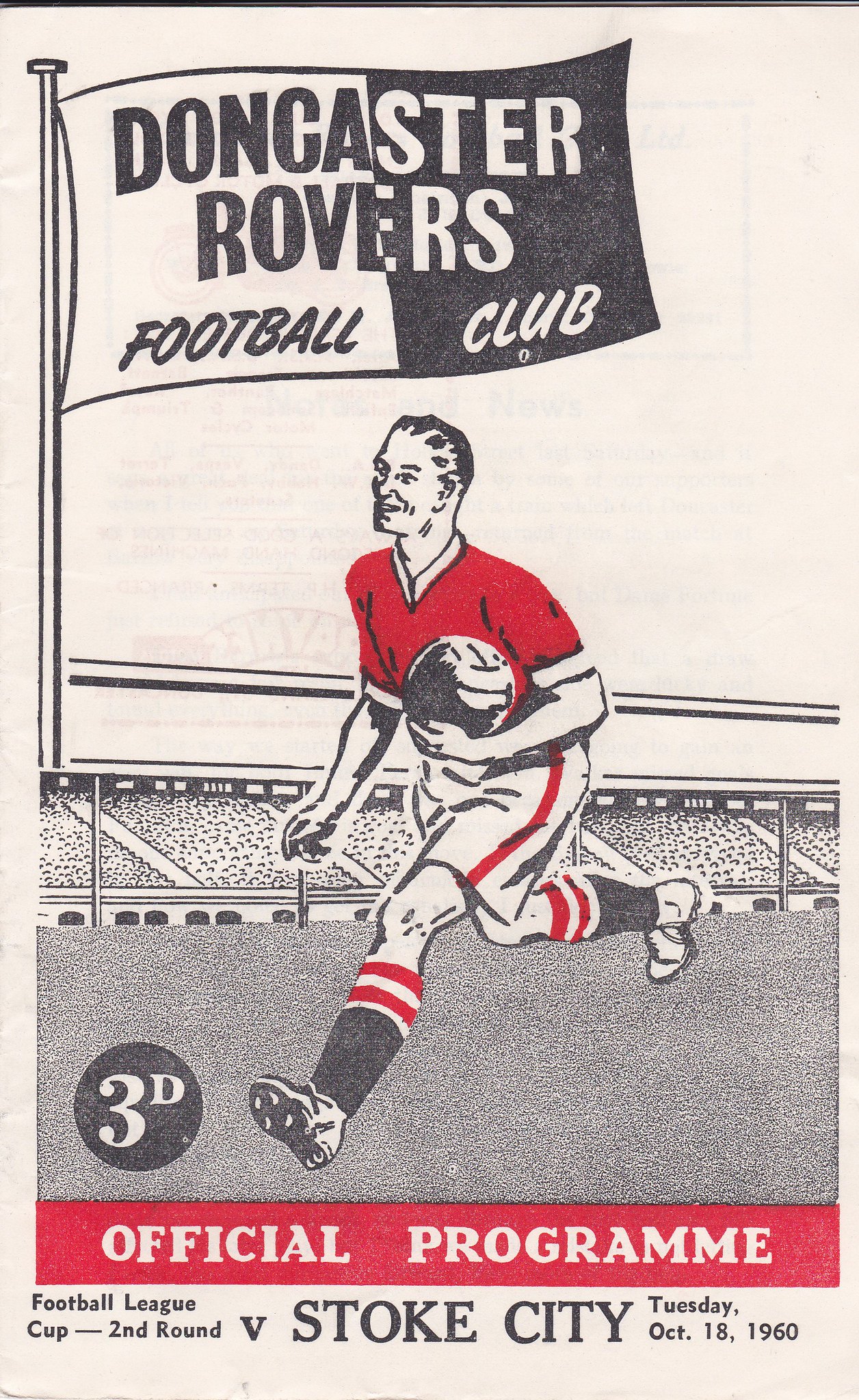This image, approximately six inches high by three inches wide, is the worn and off-white front cover of an official program from the Football League Cup second round match between Doncaster Rovers and Stoke City, held on Tuesday, October 18, 1960. The top portion of the image features a black-and-white flag divided into two halves, with "Doncaster Rovers Football Club" printed across both sides. Below the flag, a detailed graphical drawing depicts a soccer player in motion, dressed in a red jersey, white shorts with red stripes, and black socks topped with red and white stripes, holding a soccer ball in his left hand. Behind him, there's a bleacher filled with spectators and a flagpole with the flag of the club. At the player's feet is a black circle bearing the cost "3D" in white print. Beneath this, a red horizontal band showcases "Official Program" in white text, followed by "Football League Cup, Second Round, versus Stoke City, Tuesday, October 18, 1960" written in black print.